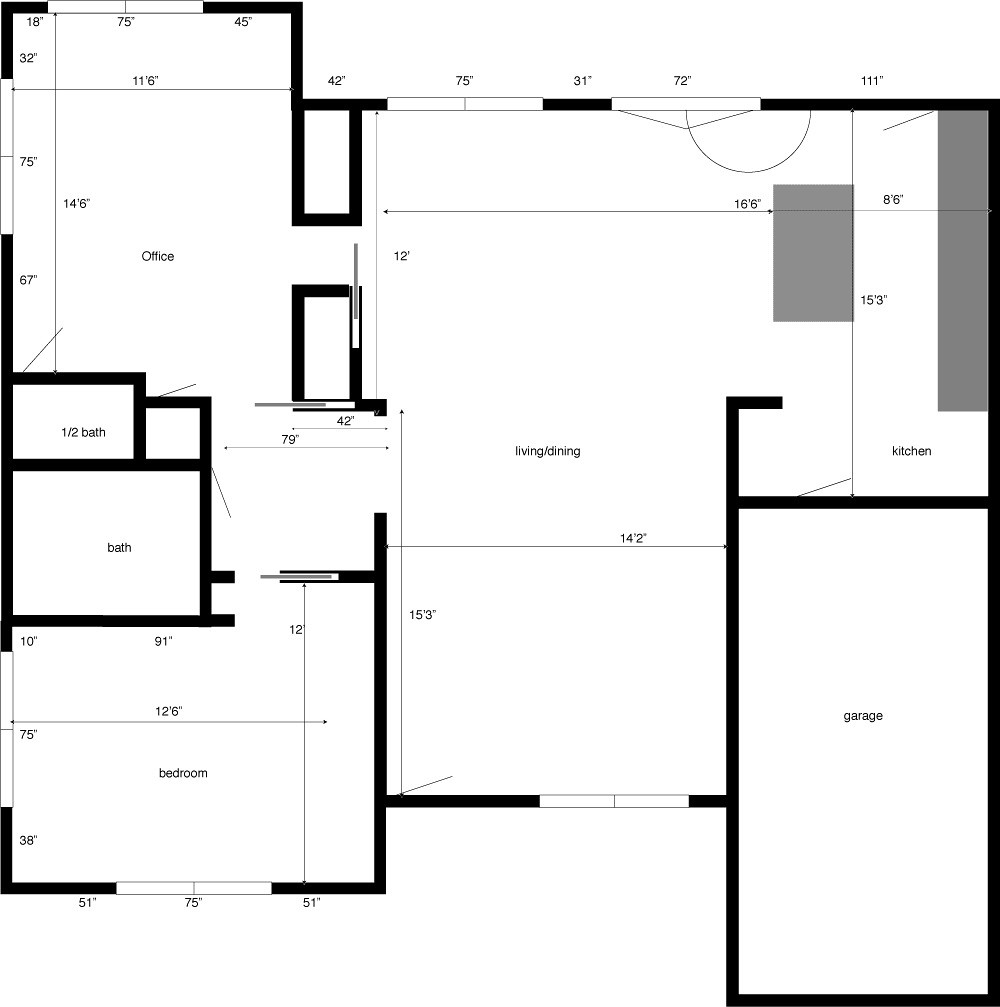This is a detailed black and white blueprint of a residential property, likely depicting the first floor of a house or perhaps a smaller dwelling. The blueprint meticulously outlines each room, complete with measurements and dimensions, except for the bathroom, half bath, and garage.

In the bottom left corner, we see a bedroom attached to both a full bathroom and a half bath. Directly above this bedroom, occupying the upper left corner, is a spacious office that opens into a centrally located living and dining room. To the right of the dining room, the blueprint reveals a well-proportioned kitchen. 

Adjacent to the kitchen, positioned below it in the layout, is an attached garage. To the left of the garage, there is an empty foyer, which provides the main entryway into the home.

The blueprint provides a comprehensive overview of the layout and functional flow of the house, highlighting the interconnectedness of these principal areas.